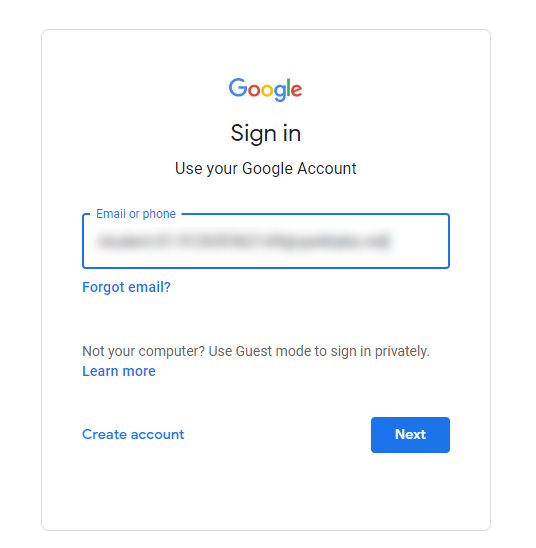Image Description: 

The image features the login page for a Google account. 

At the top, centered, the iconic Google logo is prominently displayed, with each letter in vibrant, distinct colors: the "G" in blue, "o" in red, "o" in yellow, "g" in blue, "l" in green, and "e" in red. 

Below the logo, in black text, it states "Sign in." 

Further down, it instructs users to "Use your Google Account," also in black text.

The central part of the image showcases a white rectangular input field outlined in blue. Inside this field, in light blue text, it reads "Email or phone," though the actual input is blurred out, obscured by a black blur to protect the user’s privacy.

Below this input field, aligned to the left in blue text, it says "Forgot email?” followed by a blue question mark.

Below the input field section, in black text, a sentence reads "Not your computer?" and follows with "Use Guest mode to sign in privately."

Further down, in blue text, it offers a link to "Learn more."

At the bottom of the image, in blue text, it provides an option to "Create account."

Lastly, a prominent blue rectangular button is displayed with the word "Next" in white, urging the user to proceed with the sign-in process.